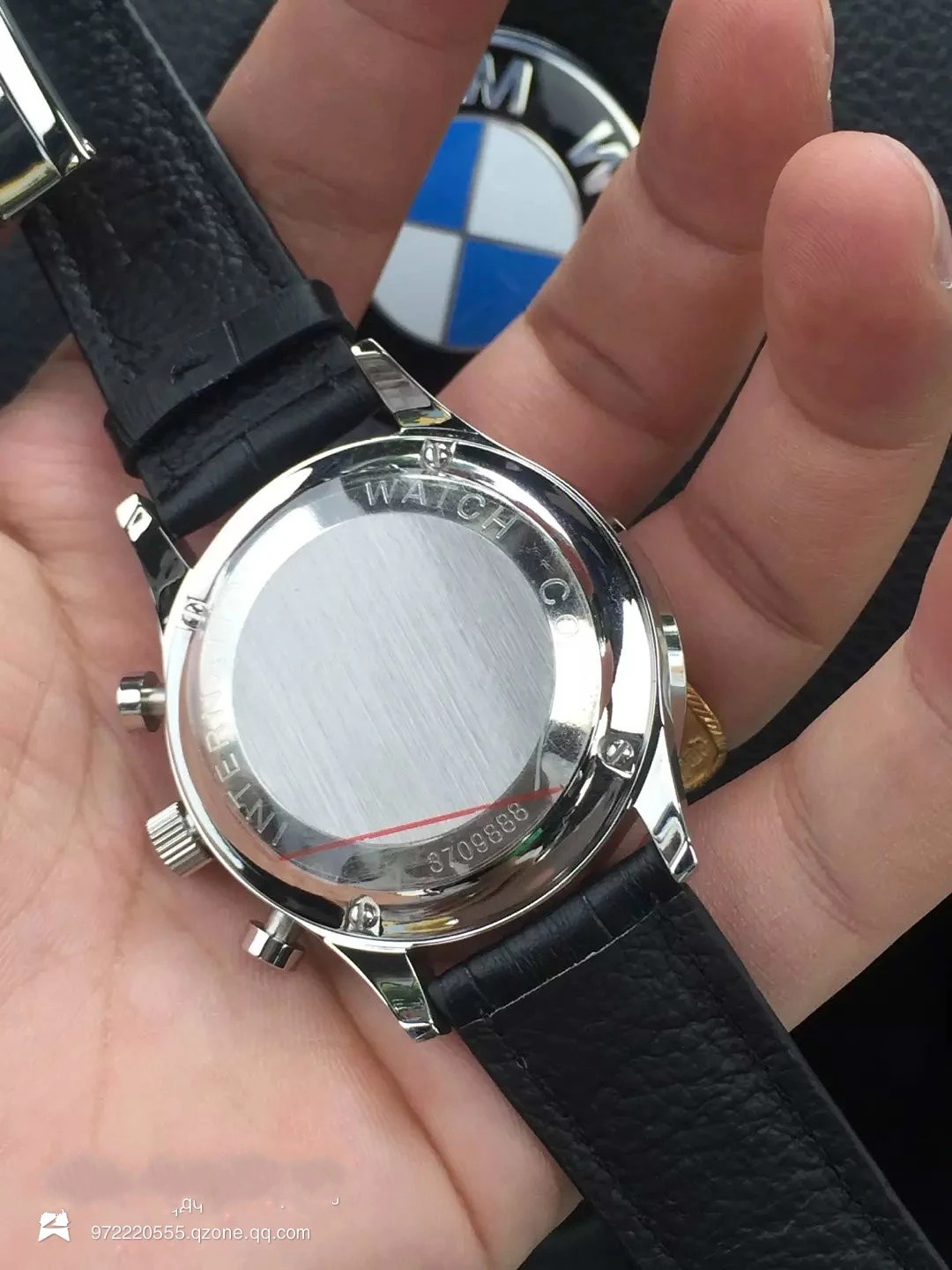The image features a close-up of a person's right hand, smooth and clean with well-trimmed nails, holding a watch with a black leather strap. The watch's silver back is facing the camera, revealing partial text: “INTER” and “watch,” along with a number sequence, 'S709888'. The hand, adorned with a gold band on the ring finger, is positioned in front of what appears to be a BMW steering wheel. The BMW logo is partially visible in the background, showing the distinctive blue and white triangles that form the emblem, along with the letters 'M' and 'W'. The combined clues suggest the photo was taken inside a BMW vehicle.